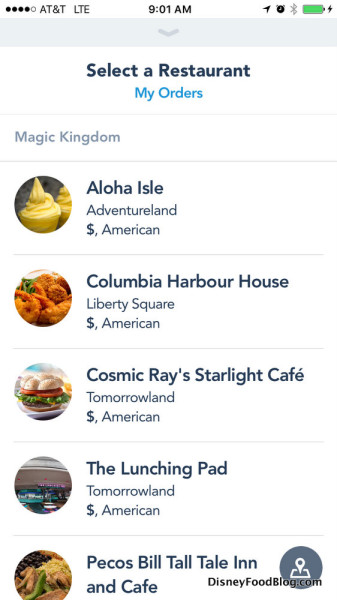The image features a user interface with a white background and a gray border near the top, including a small drop-down arrow that suggests it can be expanded. At the top, there are four black dots, with one unfilled dot beside the text "AT&T LTE." Centered prominently at the top is the time "9:01 AM" in bold font. The upper right corner displays icons for a right-diagonal arrow, an alarm clock, a Bluetooth symbol, and a fully charged green battery with a charging icon.

Below the top bar, the heading "Select a Restaurant" appears in navy font, with a lighter blue, clickable link labeled "My Orders." Beneath this section, the text "Magic Kingdom" is presented in gray. A list of restaurants follows, each with detailed descriptions:

1. **Aloha Isle, Adventure Land** - "American" cuisine, indicated by a dollar sign, featuring a yellow ice cream icon.
2. **Columbia Harbor House, Liberty Square** - "American" cuisine, noted with a dollar sign, displaying icons of fried shrimp and chicken.
3. **Cosmic Ray's Starlight Cafe, Tomorrowland** - "American" cuisine, symbolized by a dollar sign and an icon of a burger.
4. **The Launching Pad, Tomorrowland** - "American" cuisine with a dollar sign.
5. **Pecos Bill Tall Tale Inn and Cafe** - Additional information provided by DisneyFoodBlog.com is noted at the bottom right corner.

This organized layout provides detailed information about available dining options in the Magic Kingdom.